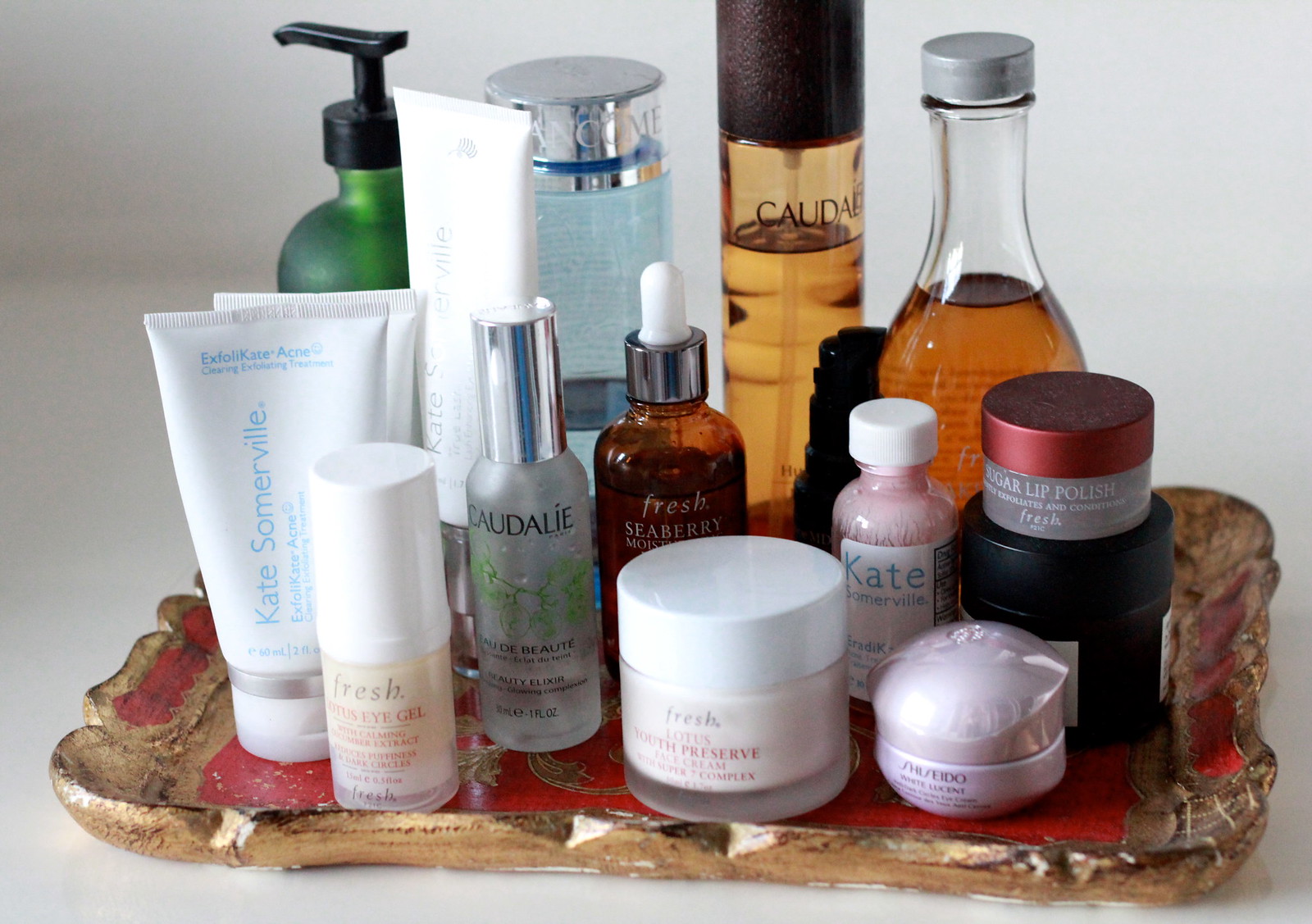This vibrant color photograph captures an artful still life composition, showcasing an elegant assembly of beauty items meticulously arranged on a luxurious tray. The tray, adorned with intricate gold embellishments, shows signs of age with chipped corners, suggesting a cherished, well-used piece. It rests against an indistinguishable expanse of pure white, blending seamlessly with both the background and the surface it sits upon, drawing focus to the tableau of products.

The display on the tray features an assortment of skin creams, perfumes, and serums, each housed in containers of various shapes and designs. The palette of the items ranges from light yellow, green, white, and peach to vivid pink, red, and orange, creating a visually pleasing contrast. Among them, a tall bottle filled with a yellowish liquid stands out slightly right of center, becoming the focal point of the image. This particular bottle, capped with a silver top, radiates elegance and sophistication.

Additional highlights include slender glass bottles and sleek tubes, some crowned with polished silver caps, others with stark white tops, one of which features a practical pump dispenser. Intricate text scrolls around the bottles and tubes, adding a layer of detail and authenticity to the composition. These exquisite items, ranging from perfumes to serums, epitomize feminine beauty products, delicately poised in this refined still life arrangement.